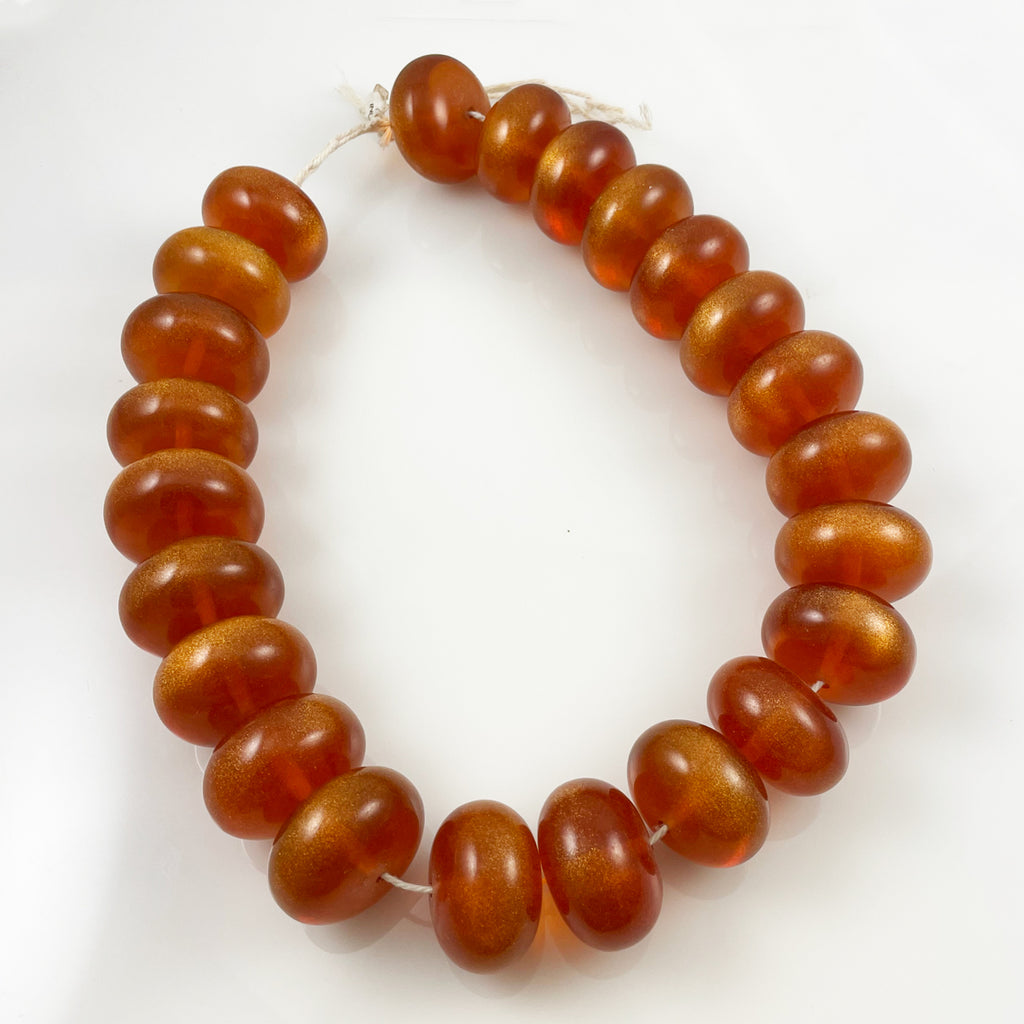The image showcases a detailed and close-up view of a beaded necklace or bracelet, centrally placed against a white background. The string running through the beads is white, likely made of cotton. The beads themselves are primarily amber in color, with a honey-like, semi-translucent quality that exhibits a slight interior glow, suggesting they might shine more brilliantly in sunlight. They are elliptical, bulging, and flattened at the top, resembling vintage jewelry. The beads also vary in size, with the largest positioned at the bottom of the image. The beads seem almost fluid, as if they are oblong circles of solidified liquid, and have a shimmering, yellowish-gold glitter embedded within. The overall appearance is clear, bright, and reminiscent of vintage jewelry, possibly invoking thoughts of smooth, candy-like butterscotch pieces.